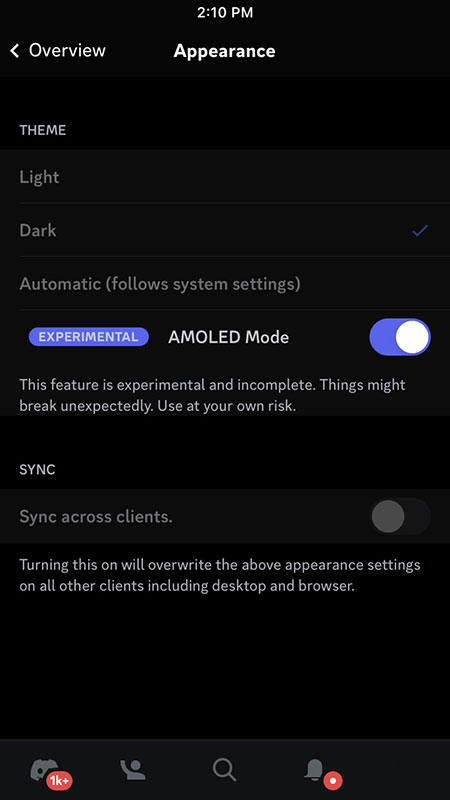Screenshot of a smartphone displaying the Appearance settings menu at 2:10 PM. The background is entirely black, and the status bar at the top shows no icons. A row of icons at the bottom features a gaming icon with "1K" in red, a person waving, a search icon, and a bell icon with a red notification circle.

The main screen area begins with "Overview" on the left and "Appearance" centered, both in white text. Below this, the "Theme" section lists "Light" and "Dark" options, with "Dark" highlighted by a blue check mark. The "Automatic" option follows, accompanied by the note "(Follow System Settings)".

Next, in a blue rectangular oval, appears the "Experimental" category, featuring "AMOLED mode" with a blue oval and a white dot indicating it is turned on. A warning below notes that this feature is experimental and may cause issues, advising caution.

Lastly, the "Sync" section explains "Sync across clients" with a gray oval and circle, showing the feature is off. A note clarifies that enabling this will override the appearance settings on all clients, including desktop and browser.